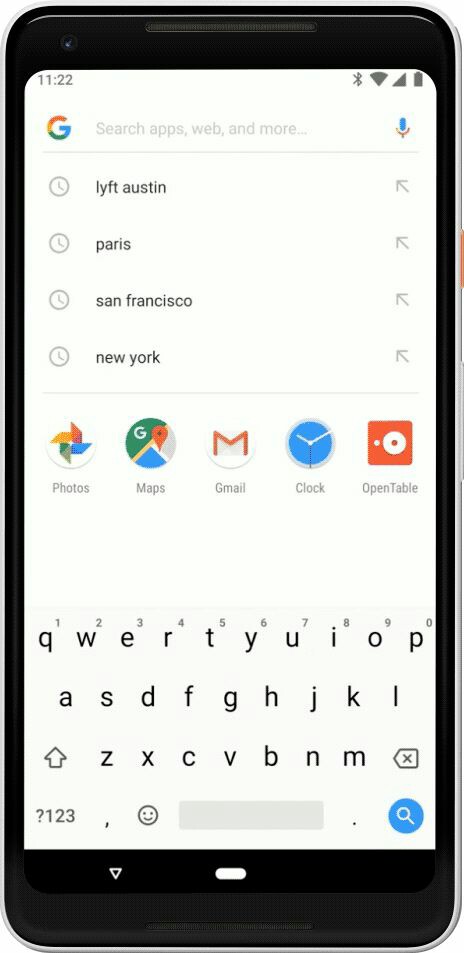The image depicts a smartphone's screen with various features and applications visible. The main display shows a predominantly white background with black text, featuring multiple options that appear to have been selected previously. The text is rendered in a moderately sized font that is easily readable. 

At the top of the screen, basic phone notification symbols are displayed. On the top left, the current time is 11:32. On the top right, there are icons indicating signal strength, Bluetooth connectivity, and battery status. 

Towards the bottom, a standard QWERTY keyboard is visible, equipped with typical keys and a magnifying glass icon on the bottom right, likely representing the search function. 

In the middle section of the screen, various app icons are arranged, including Photos, Maps, Gmail, Clonk, and OpenTable. Most of these icons are circular, except for the OpenTable app, which is presented in a square shape.